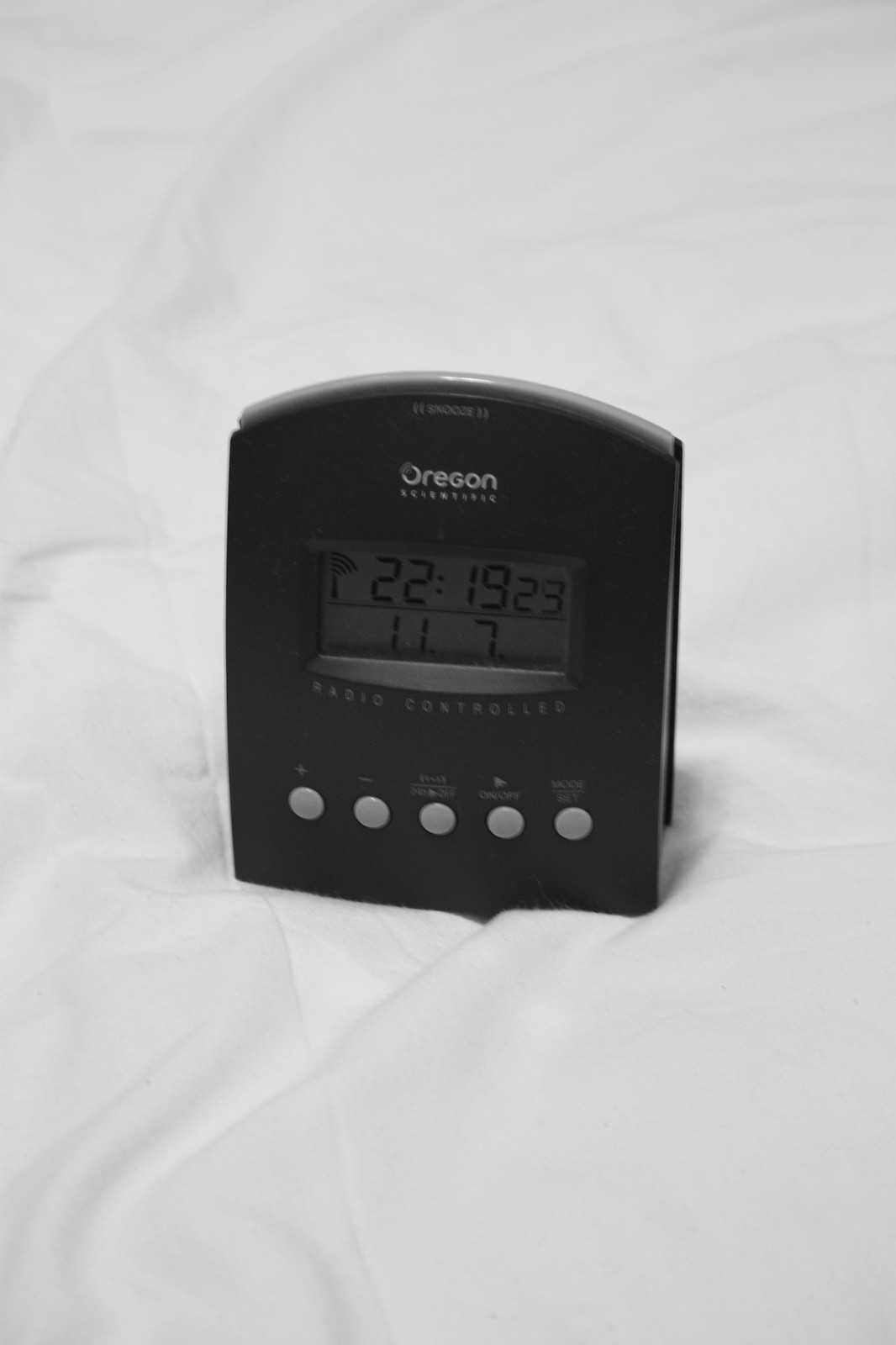This image showcases a sleek, compact clock, likely a radio-controlled digital device. The clock is predominantly black with a rectangular gray screen displaying the time in black digits, reading "22:19" hours and "23" seconds. Below the time, the display indicates the date as "11" and "7," possibly signifying November 7th. Beneath the date display is the text "Radio Controlled" indicating its synchronization feature with radio signals for accurate timekeeping. 

The clock features five small gray circular buttons underneath the screen, labeled with various functions, including a plus sign, minus sign, an on/off button, among others that are not clearly legible. At the top of the device, the brand name "Oregon" is subtly printed in a grayish-white hue. The background setting is a white sheet, slightly wrinkled, providing a clean and minimalist ambiance to the photograph.